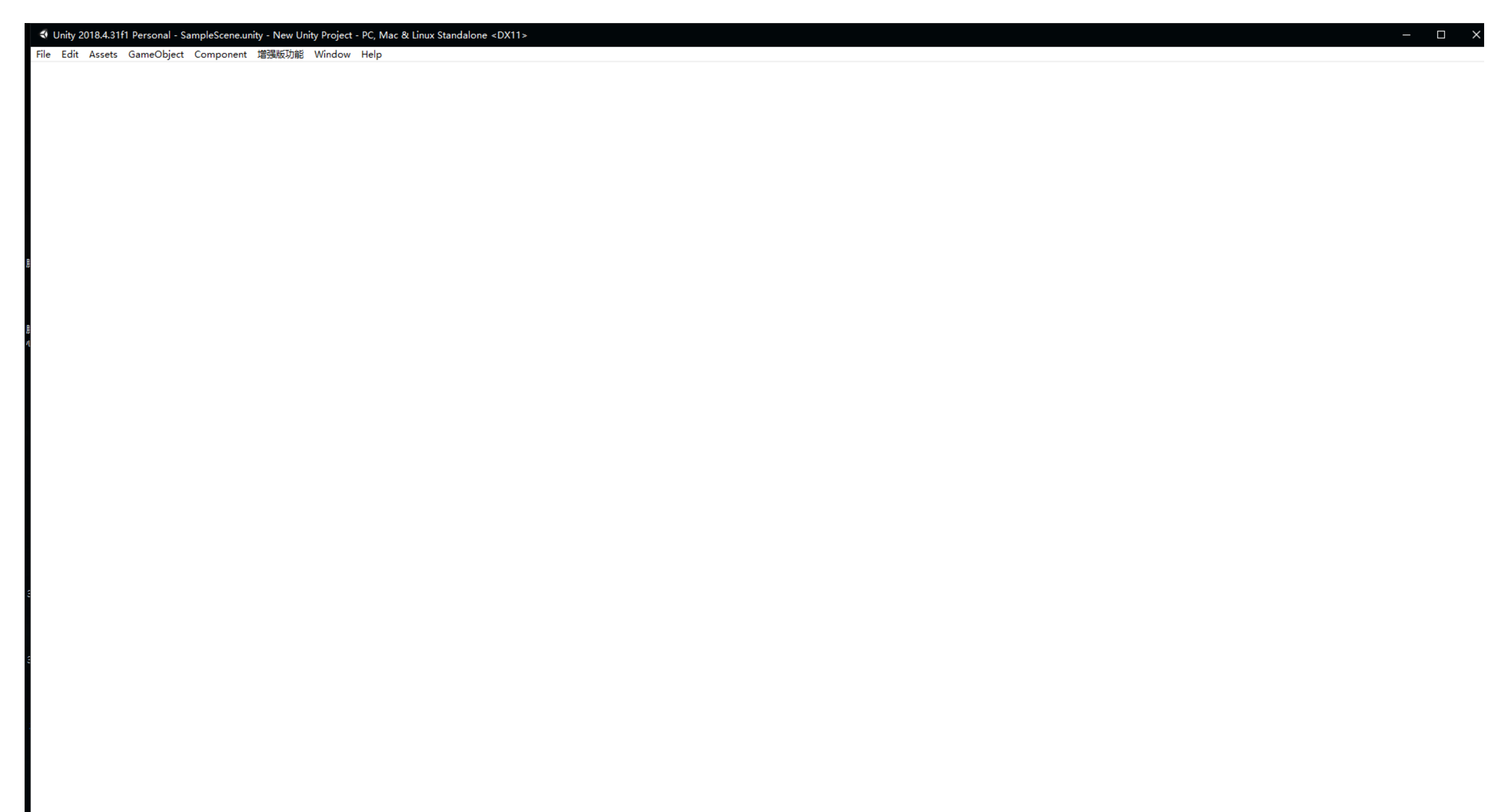This image is a screenshot of the Unity Editor interface. The main screen appears to be blank, but a black border outlines the edges. At the top of the screen, there is a black bar displaying text that reads: "Unity 2018.4.31f1 Personal" followed by "Sample Scene - New Unity Project - PC, Mac & Linux Standalone <DX11>". Below this bar, the menu options "File," "Edit," "Assets," "GameObject," "Component," "[Chinese text]," "Window," and "Help" are visible. On the left side of the top bar, the typical window control buttons are present: the minimize button, the restore down button, and the close button.